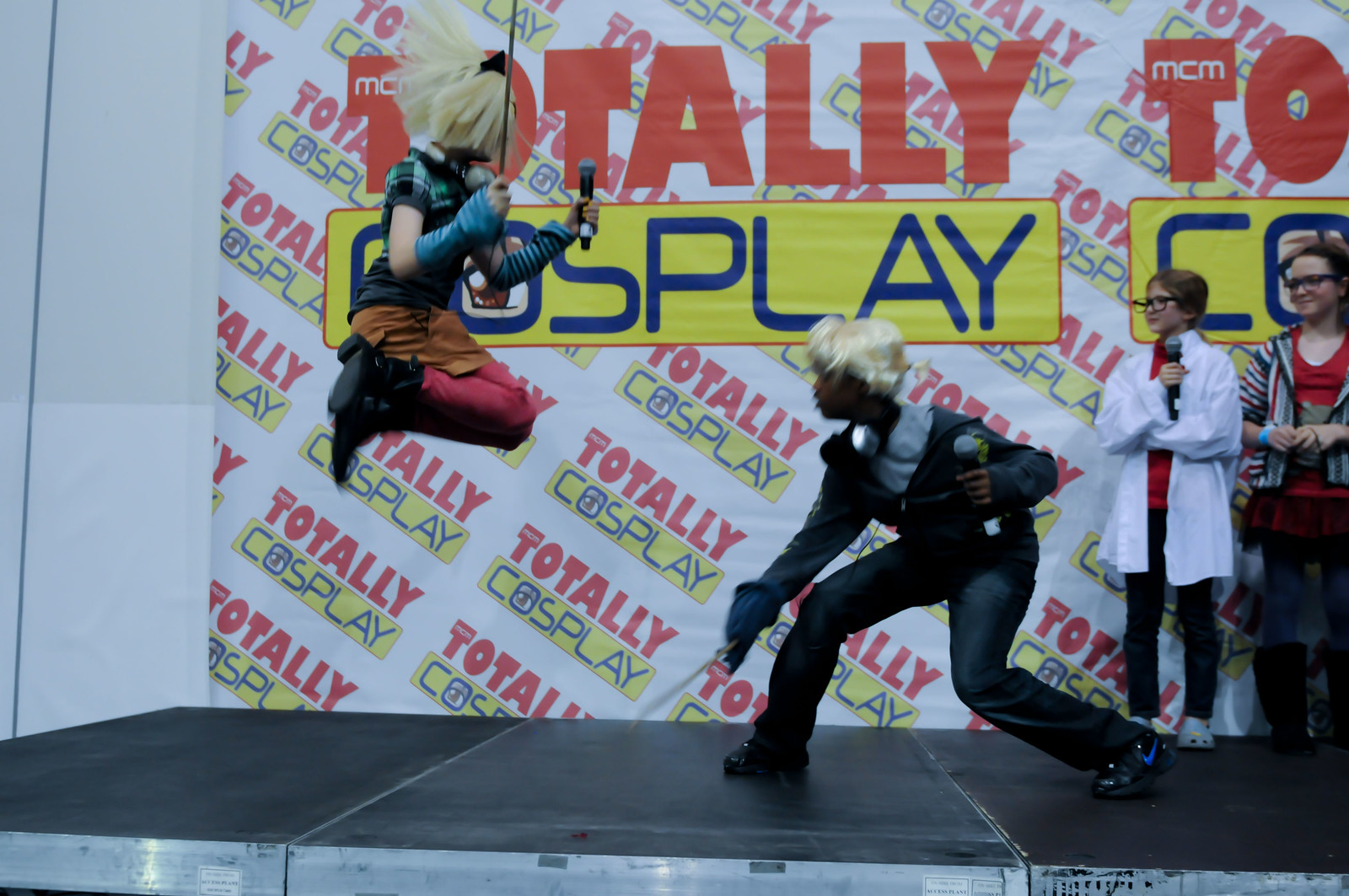The image shows a lively scene at a cosplay event, captured in full color. There are four young participants on a black stage, positioned against a white background repeatedly adorned with the phrase "Totally Cosplay" in red and yellow diagonal prints. At the center of the action, one performer with cropped whitish-blonde hair, blue gloves, a brown skirt, pink leggings, and black boots is caught mid-air, holding onto a black wire with their hair flying and legs tucked beneath them. 

Below this airborne performer, another character with short blonde hair, dressed in a dark long-sleeve shirt and pants, kneels and looks up at the jumper, engaging dynamically in the scene. Both are holding microphones, suggesting they are performing or presenting. To the right, two other participants are partially visible. One girl with red hair and huge glasses wears a white lab coat, likely portraying a scientist, and holds a microphone. Beside her stands another person in a red shirt with a multicolored sweater, though only partially in the frame. The entire scene is buzzing with energy, highlighting the creativity and enthusiasm characteristic of cosplay events.